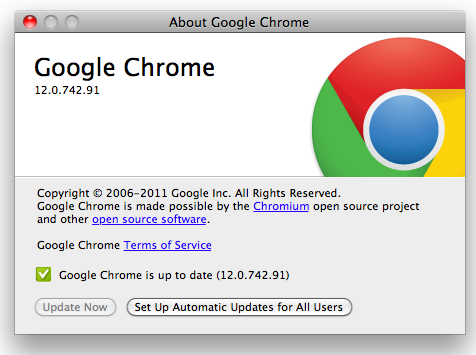A detailed view of an Apple Safari browser window displaying the Google Chrome update details. The title bar at the top of the window reads "Google Chrome," with a single red close button on the far right. On the upper right-hand side of the window, the familiar Google Chrome icon is visible, characterized by its red, green, and yellow segments encircling a blue sphere at the center. Beneath the icon, the version number "Google Chrome 12.0.742.91" is prominently displayed.

The section below the version number is filled with legal information stating: "Copyright 2006-2011, Google Inc., All rights reserved. Google Chrome is made possible by the Chromium open-source project," with "Chromium" hyperlinked in blue text, along with a mention of "other open source software" also highlighted in blue. There's a notable critique of this claim, pointing out the inaccuracy that Google Chrome itself is not an open-source browser.

Furthermore, the update status includes a green check mark indicating that "Google Chrome is up to date" with the same version number, "12.0.742.91," listed again. Options regarding updates show a grayed-out "Update Now" button and a suggestion to "set up automatic updates for all users.” The overall context indicates that this is likely an update installer for Google Chrome, with commentary disputing the open-source claim.